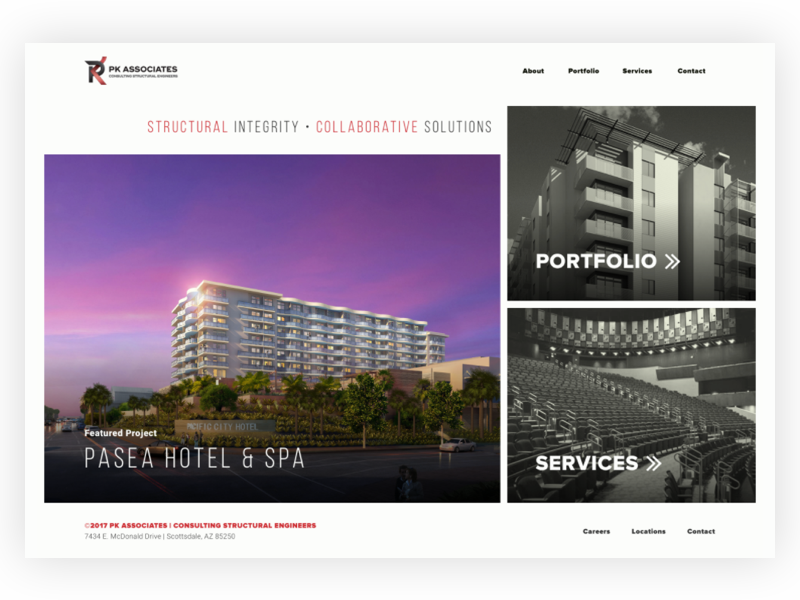This detailed caption accurately represents the elements described in the image for PK Associates:

---

The image features the logo of PK Associates prominently placed in the upper left-hand corner, accompanied by the company's name "PK Associates" directly below it. A company slogan or tagline is also situated beneath the name, though it is not specified. To the right, bold black lettering displays the headings "Portfolio," "Services," and "Contact."

Below these headings are three images arranged horizontally. The largest image, located on the left side, depicts a hotel under a purple sky framed by trees and balconies. This image is overlaid with text in red and white. "Structural Integrity" and "Collaborative Solutions" are split by a bullet point, emphasizing the firm's focus on both aspects. Additionally, the upper left corner of the hotel image features the phrase "Speech to Project" in white text, and the name "Paseo Hotel and Spa" is prominently mentioned. Beneath this image, there is a copyright symbol followed by "PK Associates, Vertical Consulting Structural Engineers." The address is partially visible, indicating the company is based in Scottsdale, Arizona.

Adjacent to the hotel image are two equally sized images. The first on the left illustrates an upward view of a multi-level building. The image has the word "Portfolio" in bold white letters with two arrows pointing to the right, suggesting navigation. The second image, on the right, shows an auditorium with tiered seating and strategic lighting aimed toward the front. This image features the word "Services," also in bold white letters, accompanied by two right-facing arrows, likely for navigation.

Overall, the collage of visuals and text aims to encapsulate the essence of PK Associates' structural engineering and consulting services.